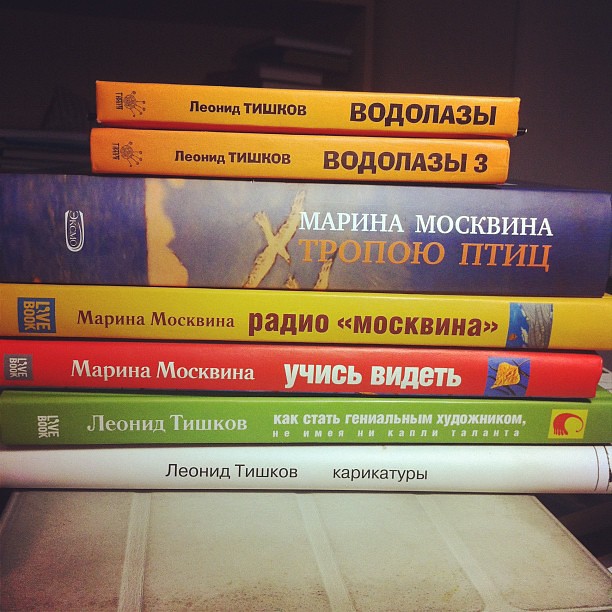This image showcases a close-up view of several books neatly stacked on top of each other, with their spines all facing the camera, revealing that they are written in Russian. Resting on a light beige tabletop, distinguished by three lines running through it, the books are set against a dark background where the outline of an additional bookshelf filled with more books can be faintly seen. The collection consists of a range of colors and sizes: the bottom book is white, followed by a green book, a red book, and a notably wide yellow book which features images of birds on its cover. On top of this is a purple book that gradually transitions to blue, also depicting seagulls and clouds. Topping the stack are two smaller orange books with distinct hand-drawn-like images of a circle with lines representing fingers and fingertips. Most of the books string from primarily two Russian authors, Marina Moskvinia and Leonid Tyskhov. The detailed text on the spines feature a mix of white, maroon, and black Russian script, with some accented by squares of different colors containing additional symbols or text.